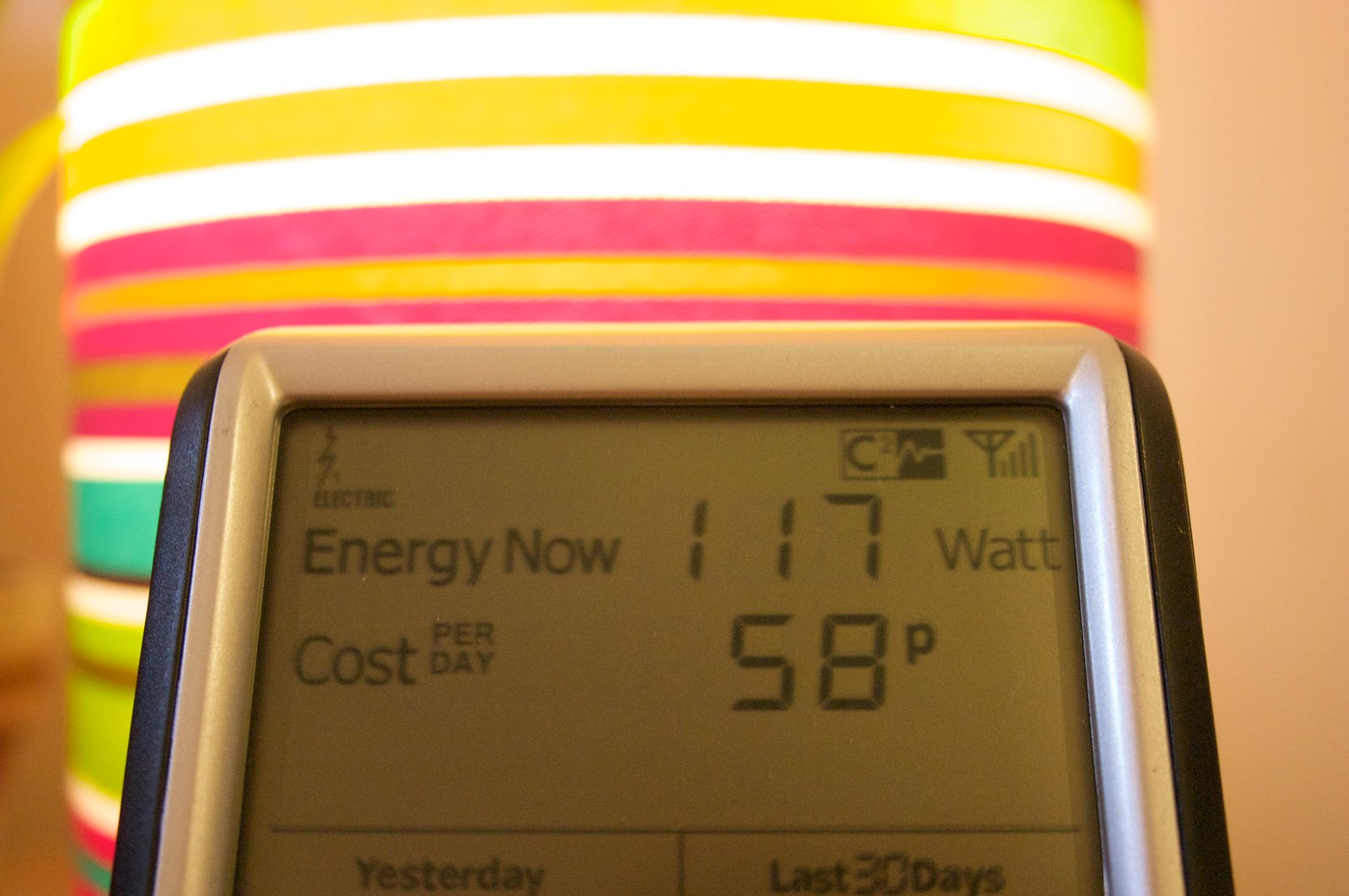A close-up view of a smart thermostat, being held up to the camera, reveals its sleek design and specific details about energy usage. The digital face of the thermostat has a gray background with black numbers and letters, providing clear readability. At the top, the display indicates that the device is connected to Wi-Fi. Below this, it informs the viewer of current energy consumption: "Energy Now: 1.7 watts" and "Cost Per Day: 58p." Additionally, it has sections titled "Yesterday" and "Last 30 Days," although the specific data for these periods is not visible in the image. The background, illuminated with a blend of yellow, white, pink, and green hues, adds a vibrant backdrop, possibly suggesting the type of lighting the thermostat is monitoring. This background lighting might be symbolic of the energy usage details displayed on the thermostat, hinting that these figures could relate to the cost of running a particular light source or bulb.